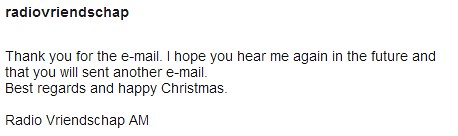The image features a simplistic design of black text on a white background, with all text left-aligned. At the very top, in bold and slightly larger letters, it reads "RADIO VRIENDSCHAP" (spelled R-A-D-I-O V-R-I-E-N-D-S-C-H-A-P). Below this, there are three lines of smaller text stating, "Thank you for the email. I hope you hear me again in the future and that you will send another email. Best regards and happy Christmas." The message concludes with a signature: "Radio Vriendschap AM."